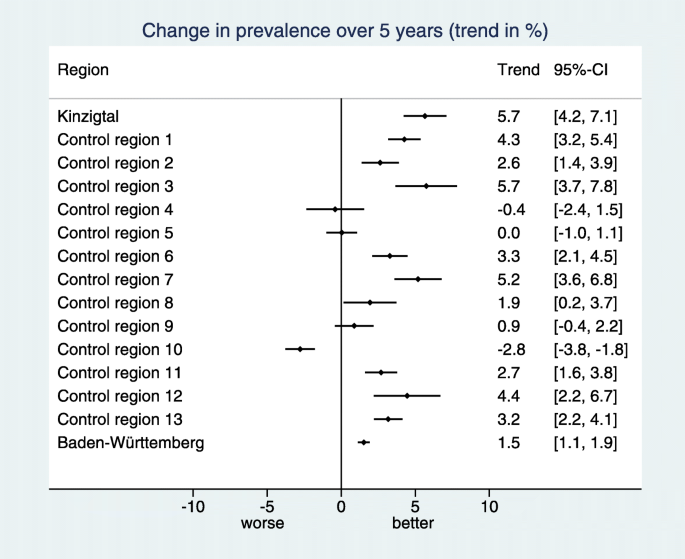The image is a detailed chart with a vertical, rectangular layout, set against a very pale light blue background. Centered within the chart, the data is presented in black text. The title at the top reads, "Change in Prevalence Over 5 Years, Trend in Percentage."

The chart is divided into several columns: "Region," "Trend," and "95% CI" (Confidence Interval). The "Region" column lists various locations starting with Kinzigal, followed by Control Region 1 through Control Region 13, and ending with Baden-Wurttemberg. Each region is associated with numerical data indicating trends over five years.

On the right side, the "Trend" column presents specific values for each region, formatted with one decimal point, flanked by brackets that display the 95% confidence intervals. The trend values include:
- Kin-Ziktal: 5.7 (4.2, 7.1)
- Control Region 1: 4.3 (3.2, 5.4)
- Control Region 2: 2.6 (1.4, 3.9)
- Control Region 3: 5.7 (3.7, 7.8)
- Control Region 4: -0.4 (-2.4, 1.5)
- Control Region 5: 0.0 (-1.0, 1.1)
- Control Region 6: 3.3 (2.1, 4.5)
- Control Region 7: 5.2 (3.6, 6.8)
- Control Region 8: 1.9 (0.2, 3.7)
- Control Region 9: 0.9 (-0.4, 2.2)
- Control Region 10: -2.8 (-3.8, -1.8)
- Control Region 11: 2.7 (1.6, 3.8)
- Control Region 12: 4.4 (2.2, 6.7)
- Control Region 13: 3.2 (2.2, 4.1)
- Baden-Wurttemberg: 1.5 (1.1, 1.9)

A vertical black line runs through the center of the chart, demarcating positive values on the right from negative values on the left, structured in increments of five. The relationship between the regions and their trends is illustrated with a horizontal line and a dot indicating the trend's position relative to the vertical line.